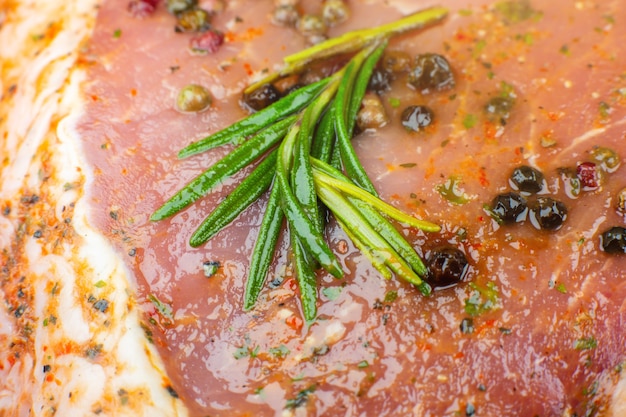This image is an extreme close-up of a piece of seared ahi tuna, showcasing intricate details of its textures and toppings. The tuna has a marbled pink center, complemented by glossy white strands, and is bordered by a seared white edge that may contain a thin layer of fat. Sprinkled across the surface are small black spheres, likely capers, adding a burst of flavor. Interspersed among these are flecks of other green and white seasonings, possibly herbs like rosemary. A sprig of a green herb lies prominently across the meat, enhancing its visual appeal. The dish appears to be garnished with a sauce that includes small red berries, emphasizing its gourmet presentation.